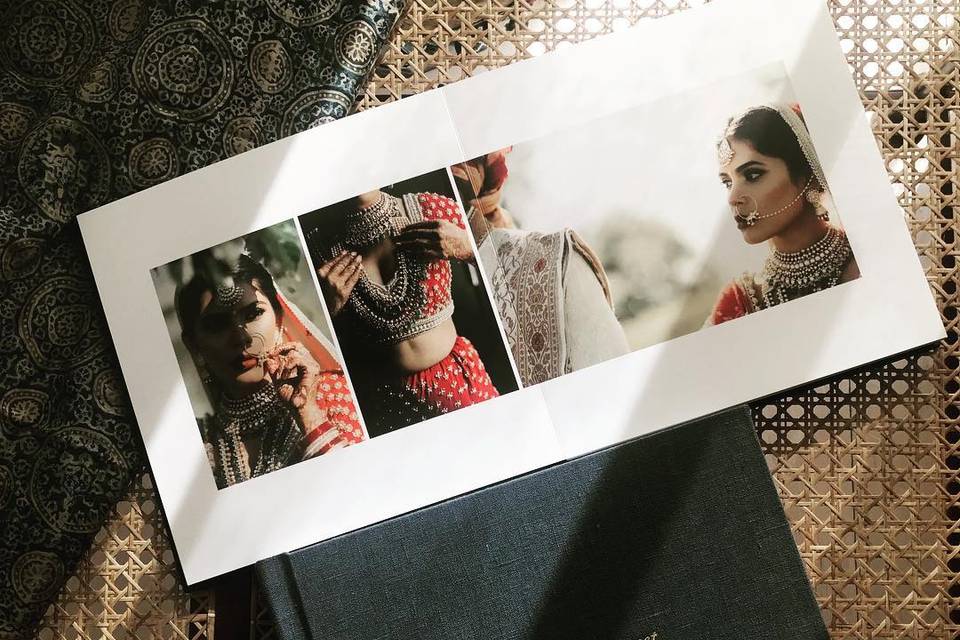This image depicts an Indian bride, likely a professional model, adorned in traditional wedding attire. The image is composed of three distinct photographs printed on a card that lies atop a wooden mat, with a blue and black book beneath it and a piece of elaborate fabric in the upper left corner. In the first photo, the bride is shown from the chest up, wearing a red sari adorned with floral patterns and intricate jewelry, including a beaded headdress, a beaded necklace, and a nose hoop with pearls. She also has red lipstick and henna designs on her hand. 

The middle photo captures the bride from the chin to her thighs, allowing a full view of her red and white designed top, her red skirt, and the detailed henna on both her hands, which are positioned in front of her. 

In the third photo, the bride is featured in the bottom right-hand corner, from the chest up, gazing to the left. The nose hoop with pearl detailing is linked to her ears by an elegant chain. Also visible in this panel is a man in traditional attire standing on the left side of the image. The entire composition rests on a textured cane background, contributing to the aesthetic richness of the scene.